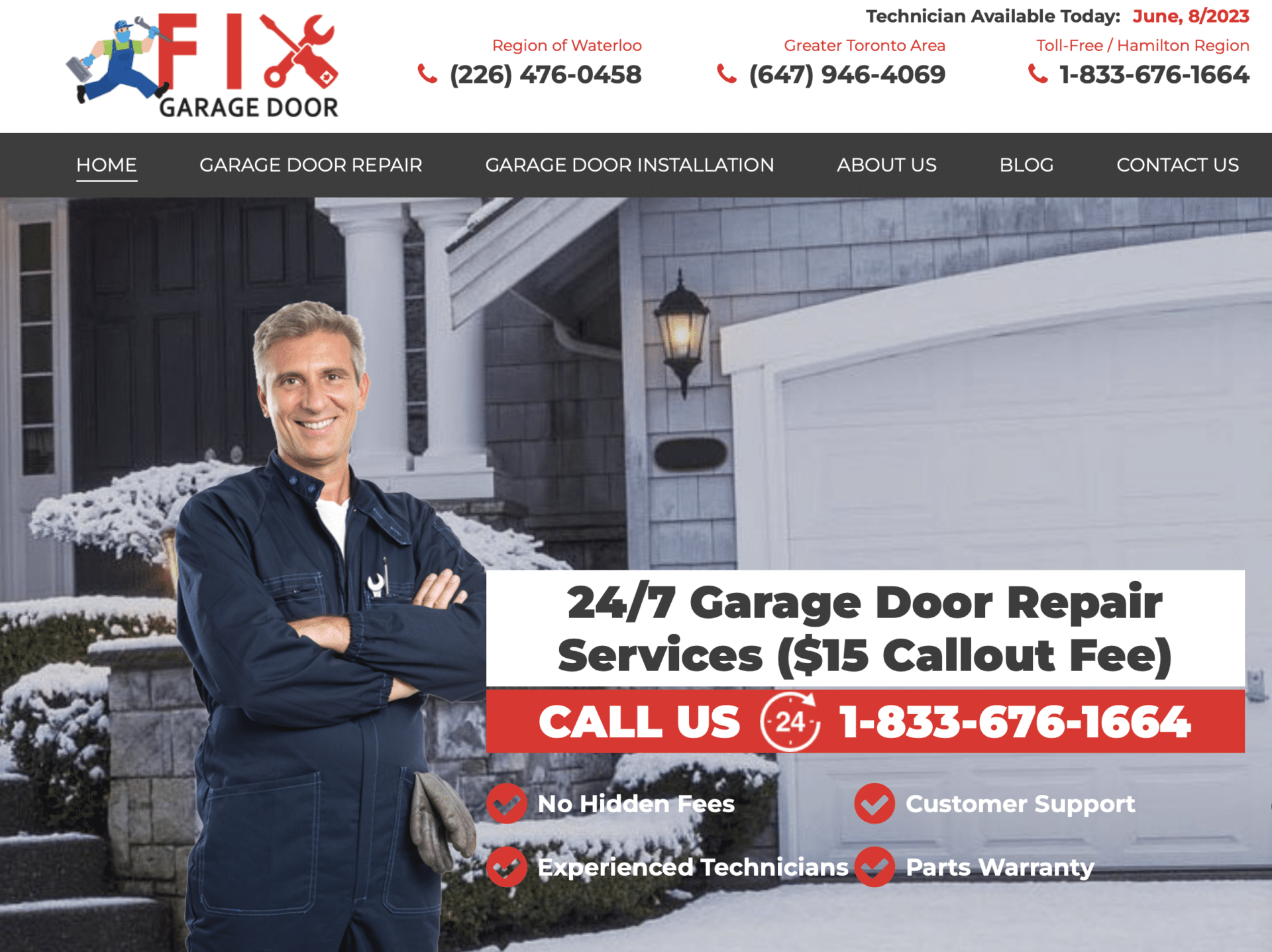The image displays a detailed advertisement for a fixed garage door service. Key elements include:

- The word "Fixed" prominently highlighted in red, emphasizing the service offered.
- An individual symbolized by the letter X, using both a wrench and a screwdriver, indicating the tools necessary for the repair.
- To the left, an illustration of a man running with a toolbox in one hand and a plumber's wrench in the other, suggesting urgency and readiness.
- The text "Region of Waterloo" in red, front and center, with associated phone numbers for the Greater Toronto Area and a toll-free number for the Hamilton region.
- Above, the phrase "Technicians available today" with the specified date, June 8, 2023, underlining the immediacy of service availability.
- Navigation options include "Home" (highlighted and underlined), "Garage Door Repairs," "Installation," "About Us," "Blog," and "Contact Us," located beneath a black bar with white text.
- On the right, an image featuring a man standing confidently in front of an elegant brick home, arms folded, smiling, dressed in a professional one-piece uniform, indicating reliability and professionalism. The garage is visible to the right and stairs leading to the main door on the left, framing the residential setting.
- A 24-7 garage door repair services box announces a $15 call-out fee.
- Below, in red and white letters, it says, “Call us 24 hours a day” with the phone number 1-833-676-1664.
- A series of service guarantees follow, each with a red check mark: "No hidden fees," "Customer support," "Experienced technicians," and "Parts warranty."

This comprehensive and visually dynamic caption underscores the availability, reliability, and comprehensive nature of the garage door repair service.